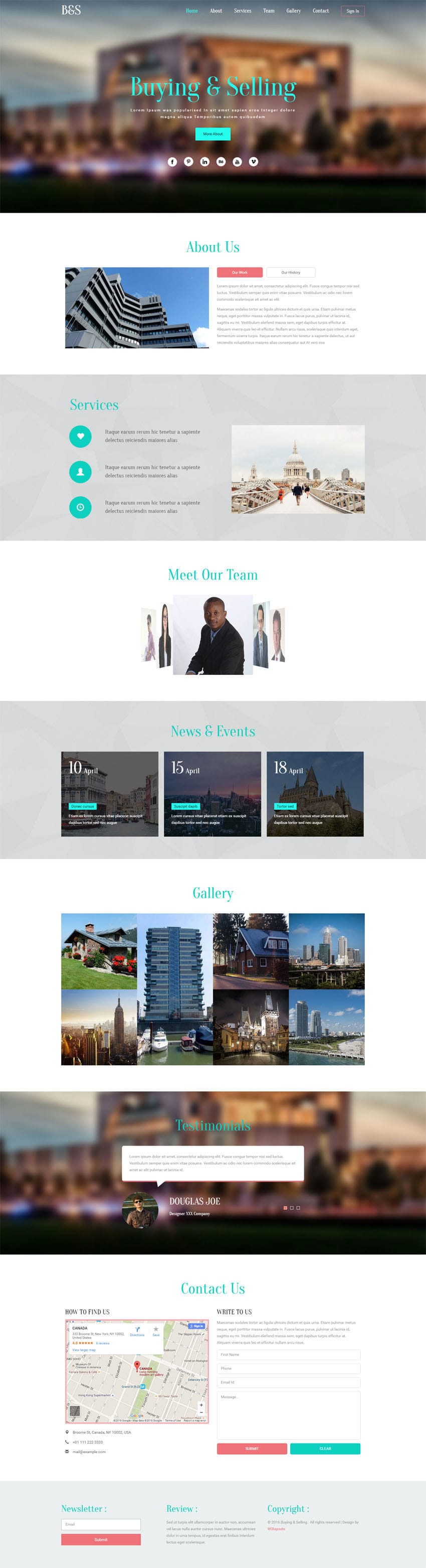This image is a detailed screenshot of a very long webpage, seemingly captured from a mobile device and then pasted into another software. The layout of the page is as follows:

1. **Header Section**:
   - At the top, there's a section titled "Buying and Selling," highlighted in blue. 
   - Underneath this title, there's a prominent blue button.
   - The background features an image of a house.

2. **About Us Section**:
   - Below the header, there's a white section with the title "About Us" in blue at the top.
   - On the left side of this section is an image of a building.
   - To the right, there's a paragraph of text that is too small to read clearly in the screenshot.

3. **Services Section**:
   - Moving down, there's a gray banner located around the center of the page.
   - This banner displays a thumbnail image of a building on the left.
   - To the right, the section is titled "Services" in very small blue letters.
   - Below this title, there are three blue bubbles, each accompanied by claims or descriptions.

4. **Meet Our Team Section**:
   - Further down, there's another white banner titled "Meet Our Team."
   - This section includes thumbnails of different employees. Each thumbnail appears clickable, allowing users to scroll through and learn more about each team member.

5. **Contact Us Section**:
   - At the bottom of the webpage, there is a section titled "Contact Us."
   - On the left side of this section is a map.
   - To the right, there is a form where users can enter their contact information to request a callback.

Overall, the page is well structured, featuring distinct sections for key information, each color-coded for clarity and ease of navigation.